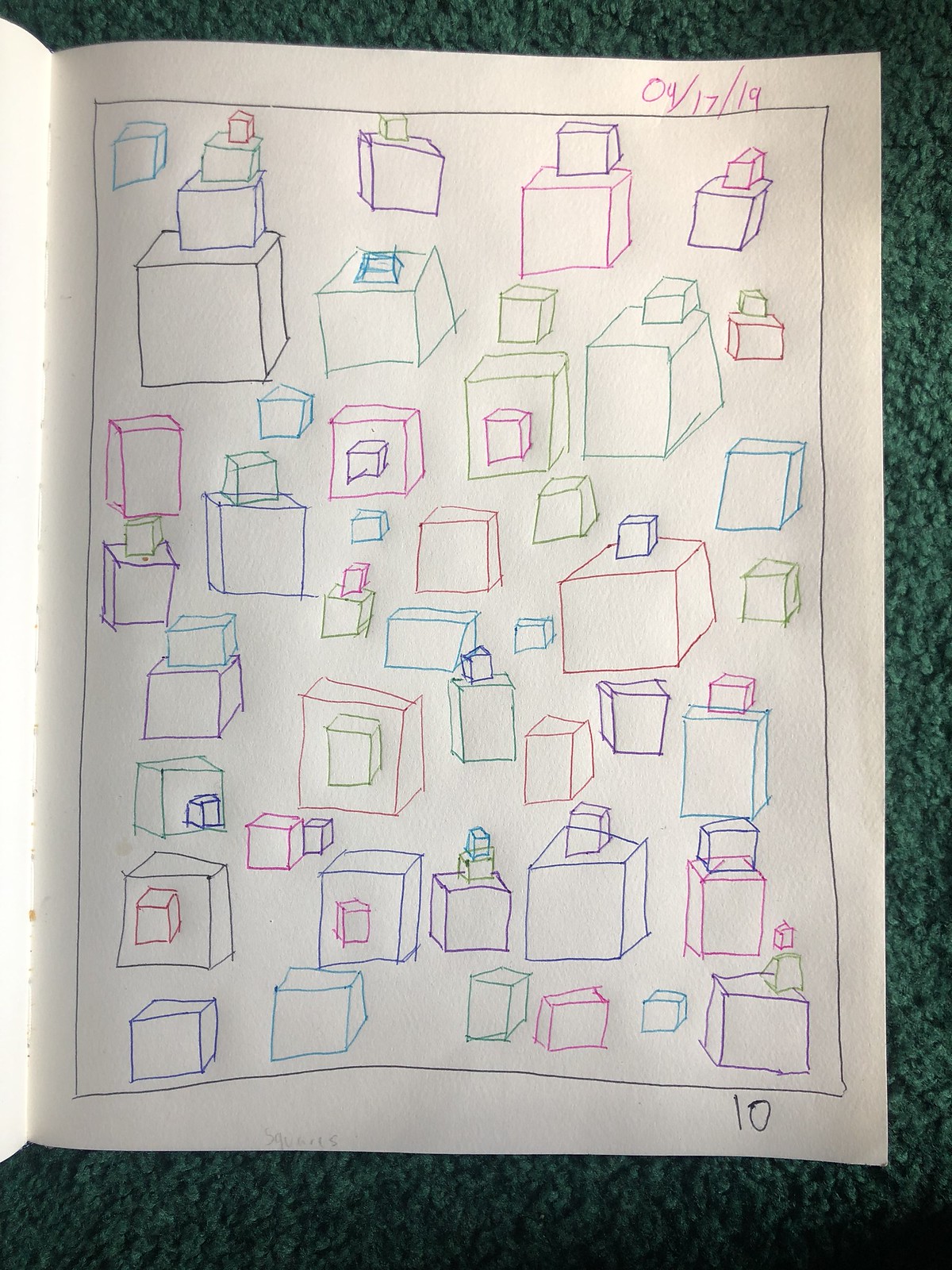The photograph, taken indoors, features a dark green carpet as the backdrop. Resting atop the carpet is an open, blank notebook, showcasing a white page with an intricate drawing. The drawing is framed by a black pen border and is dated "04/17/19" in the top right corner. Within the border, there are numerous outlined cubes of varying sizes and colors, created using different colored pens including black, green, purple, blue, red, and pink. These cubes are arranged in diverse configurations—some nested within each other, others stacked, and some standing alone. Outside the black border, in the bottom right corner of the page, the number "10" is written. None of the cubes are shaded, emphasizing their connected yet distinct forms.